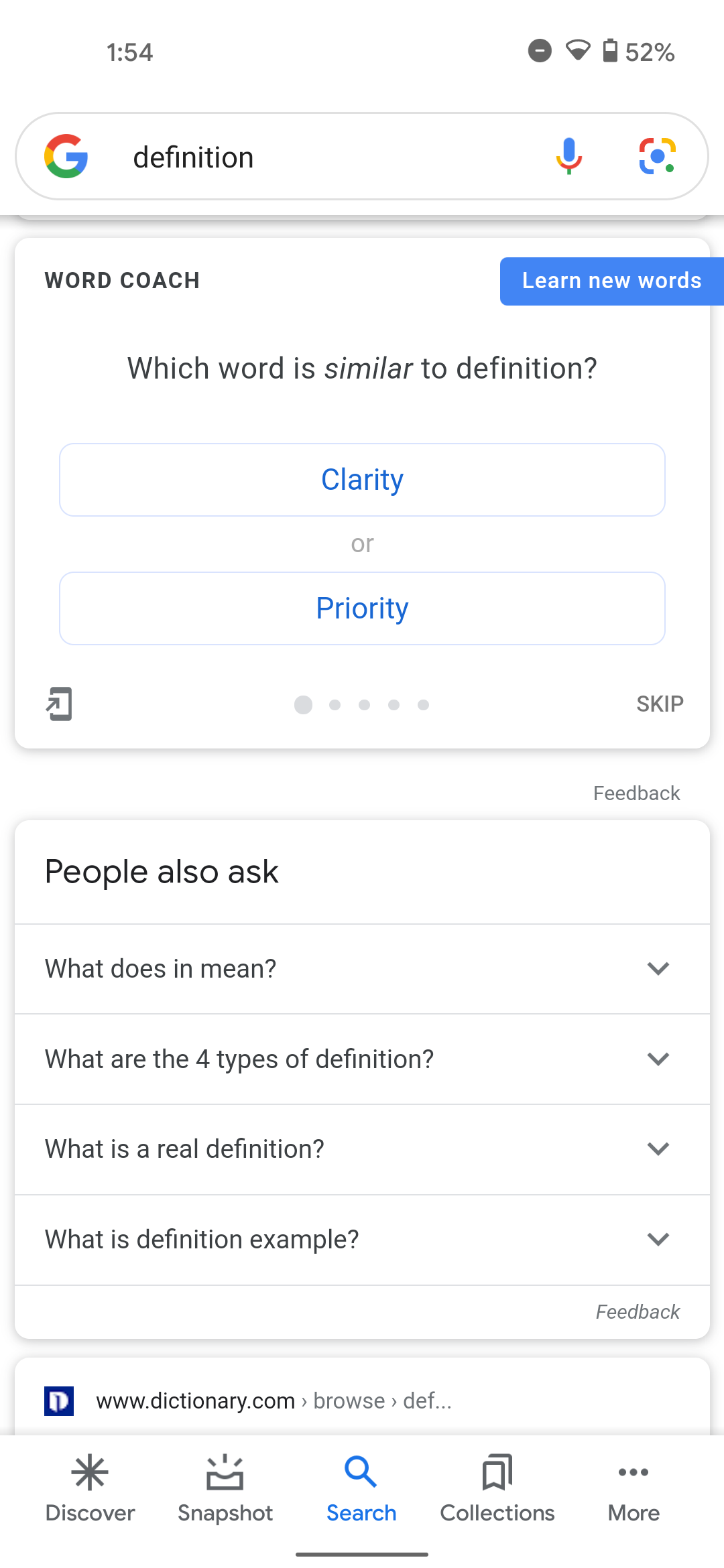In the image, the number '154' is prominently displayed alongside a Wi-Fi symbol that appears to indicate a signal strength of 52%. Adjacent to this is the Google 'G' logo, accompanied by the word 'definition'. Below these elements, there's a red, yellow, and blue square without a top. The word 'coach' is written nearby. A large blue rectangle contains the phrase 'learn new words'.

Further inspection reveals a section about determining which word is similar to 'definition'. Names like 'Lewis' appear alongside terms like 'clarity', 'priority', and a '.' symbol. Options to 'skip', to proceed to the next section, and an icon resembling a phone are also present. Additionally, there's a mention of sharing options and categories for those curious about the meaning of words, illustrated by 'what does in mean' and 'what are the four types of definition'. 

Focus is brought to 'real definition' accompanied by the phrase 'what does the definition example minty'—suggestive of more details available on dictionary sites like 'dictionary.com'. Various navigation icons like a star, a store symbol, a snapshot (half square with three lines), and a blue search magnifying glass are presented, alongside collections of three banners and a 'more' button indicated by '...'.